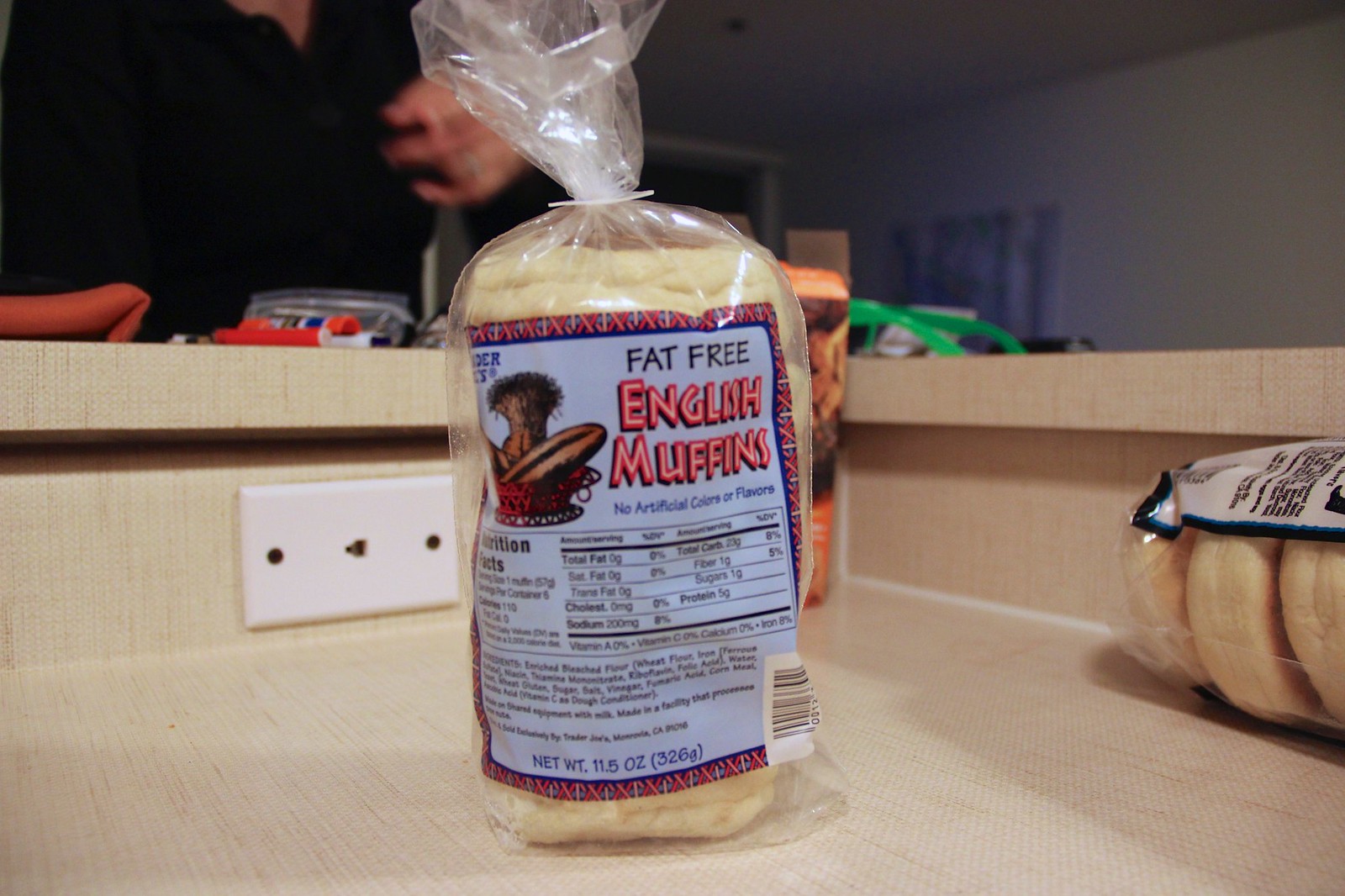The image depicts two bags of fat-free English muffins resting on a white kitchen counter. The primary focus is on a vertically standing bag of English muffins in the bottom middle of the frame, encased in a clear plastic bag sealed with one of those typical plastic clips to ensure freshness. The bag's back label, printed against a blue background, features "English Muffins" in neon red text. It also displays nutritional information, including total fat zero grams, saturated fat zero grams, trans fat zero grams, cholesterol zero grams, sodium approximately 200 milligrams, protein five grams, sugars one gram, and fiber one gram, with total carbs around twenty grams, although the exact number is difficult to read. The total net weight is labeled as 11.5 ounces or 326 grams. Below the nutritional facts, there are ingredient details and a declaration stating "no artificial colors or flavors." To the left of this text, there is an image of a toasted English muffin in a red basket, accompanied by the "Trader Joe's" logo in blue font above this picture. 

At the bottom right-hand corner of the image, partially cut off, lies another bag of English muffins, horizontally positioned, with at least three muffins visible within. Both bags are situated on a two-tier workbench with a hollowed-out section. An electrical socket is located close to the upright bag of muffins. In the background, a person with a black shirt, whose left hand is blurred in motion, stands near the counter, contributing to the dynamic setting of the kitchen scene.